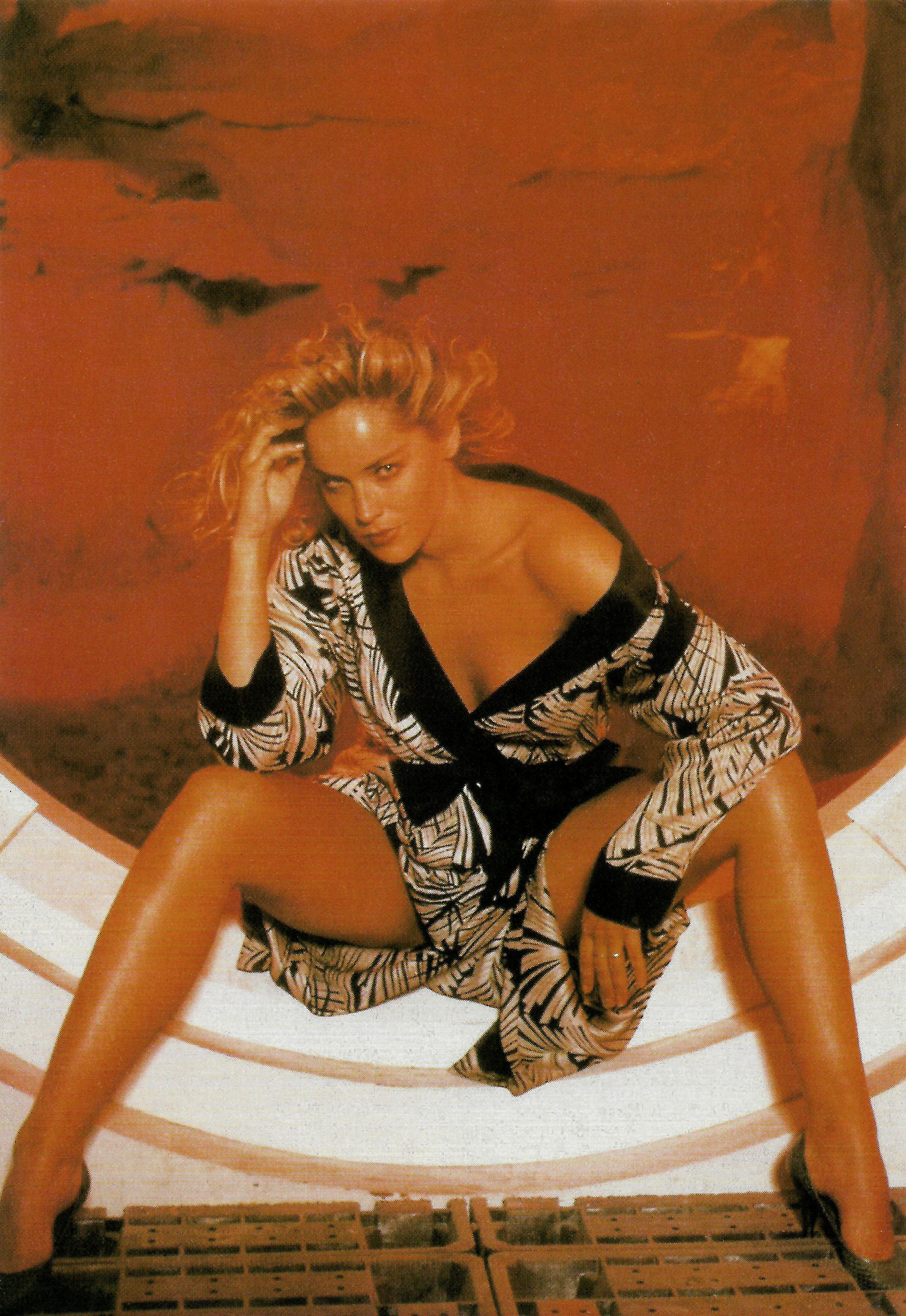The photograph captures a very tan, blonde woman, reminiscent of a younger Sharon Stone, seated in a round windowsill with only the base visible. The backdrop features a dramatic red, rocky landscape and a similarly hued sky. Beneath her, the floor consists of rectangular bricks with multiple holes, resembling a grate. The woman exudes a sensual aura, with her legs spread apart seductively, although modestly covered by her robe. She wears a simple yet striking silk robe, adorned with an intricate black and white geometric pattern, edged with a black hem at the neck, front, and wrists. Her right arm runs through her wavy blonde hair as she gazes directly at the viewer with a serious, seductive look. Completing her attire are black high-heel shoes, and a gold ring graces her left ring finger. The entire scene is bathed in a reddish-orange tint, adding to its dramatic and evocative atmosphere.